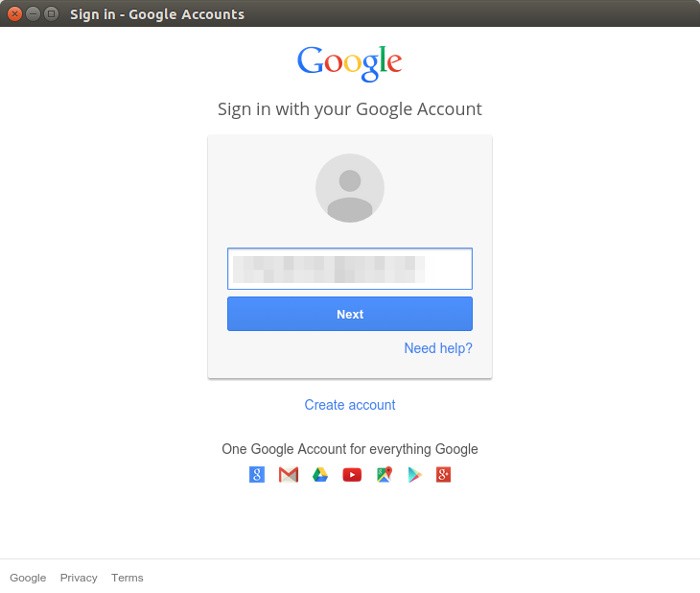The screenshot features a login interface for Google accounts, framed by a black border at the top. On the upper left side, there's a prominent red button with an X in the center, alongside two smaller gray buttons. Below the black border, large text reads "Sign in Google accounts," accompanied by the iconic Google logo, which displays a green "G," red "o," yellow "o," blue "g," green "l," and red "e".

In the middle section of the interface, there is a gray box displaying a generic profile picture placeholder. Adjacent to this, a text box is partially filled with obscured, unreadable characters. Directly below this text box is a blue button labeled "Next."

Further down, a blue hyperlink asks, "Need help?" set against a white background. Additional text below invites users to "Create account" and explains, "One Google account for everything Google." At the bottom, an array of recognizable icons symbolizes various Google services: Google Play, Google+, YouTube, Google Maps, and a blue square with a white 'G' in the center.